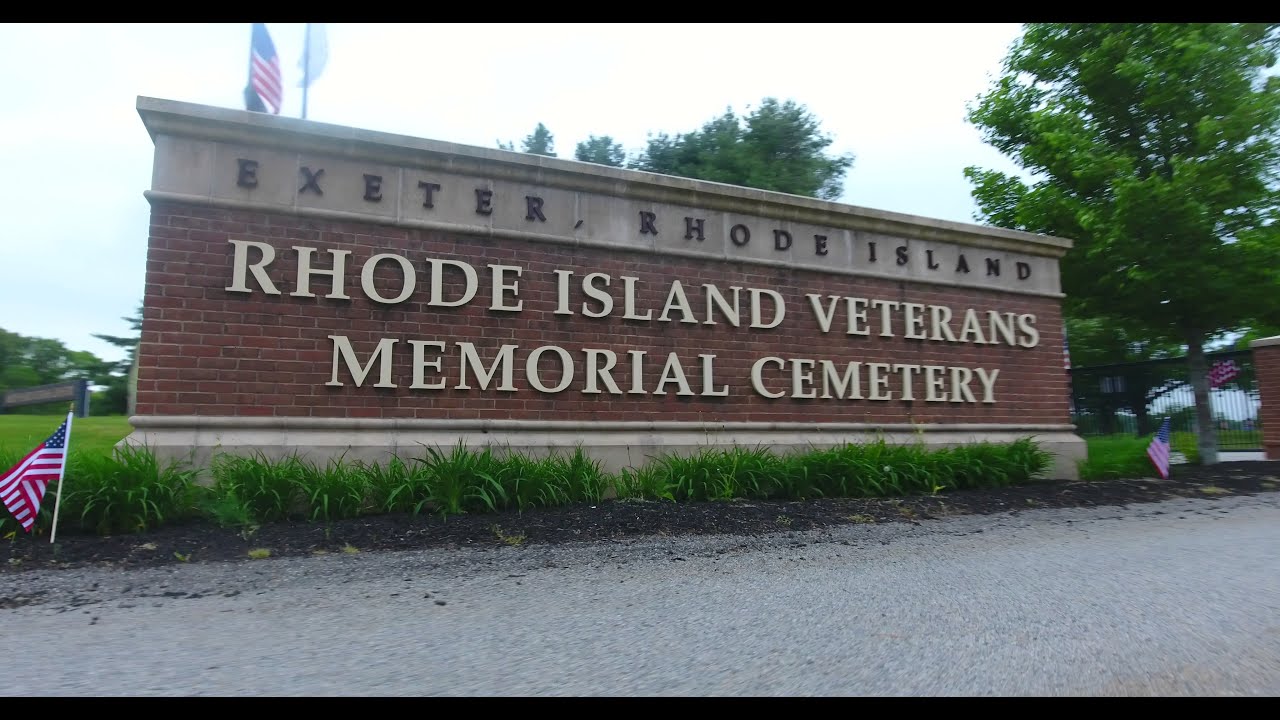The image features a prominent brick sign reading "Exeter, Rhode Island" at the top and "Rhode Island Veterans Memorial Cemetery" in cream-colored capital letters beneath. The sign is adorned with three miniature American flags: one at the top left corner and one on either side. In the background on the right, a large tree stands adjacent to an iron gate connecting to a brick pillar. The sky has a bluish-white hue, and the lighting gives a whitewash effect over the scene. Green tufts of weeds grow at the base of the sign, and a gray asphalt road is visible at the bottom of the image. The overall ambiance is serene and reflective, with additional flagpoles and trees faintly visible in the background.